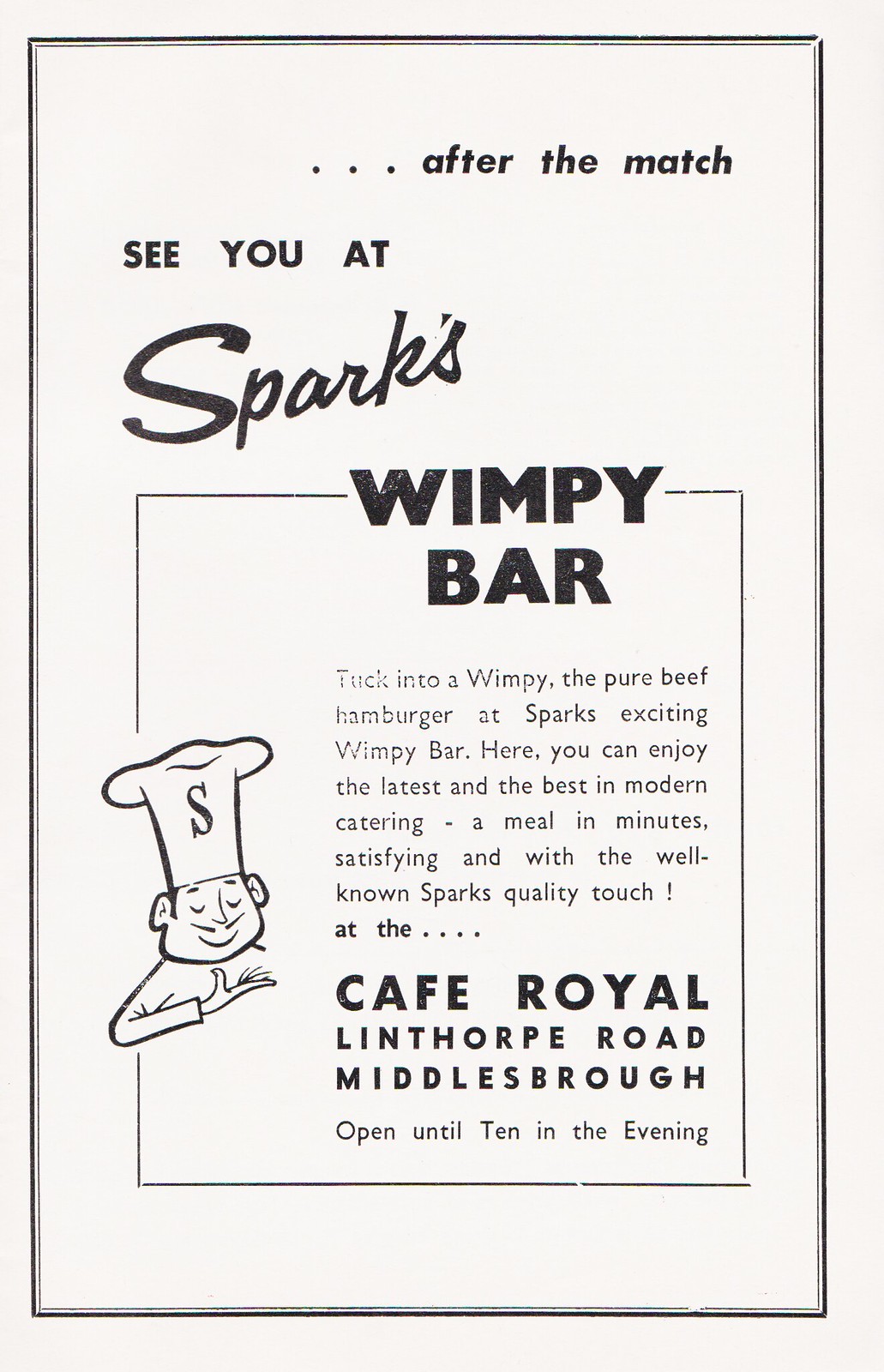This black and white flyer, vertically taller than wide, is framed by a thin, double black line. At the top, it reads, "…after the match, see you at Sparky's Wimpy Bar." The text promotes "tuck into a Wimpy, the pure beef hamburger at Spark's exciting Wimpy Bar." It highlights the convenience of enjoying "the latest and best in modern catering—a meal in minutes, satisfying and with the well-known Spark's quality touch." The flyer specifies its location at the “Cafe Royale, Lenthorpe Road, Middlesborough,” and mentions it is "open until 10 in the evening." To the left is an outline drawing of a chef with a tall white hat featuring an 'S' and a thin, upturned mustache, with his right hand raised to his chin.